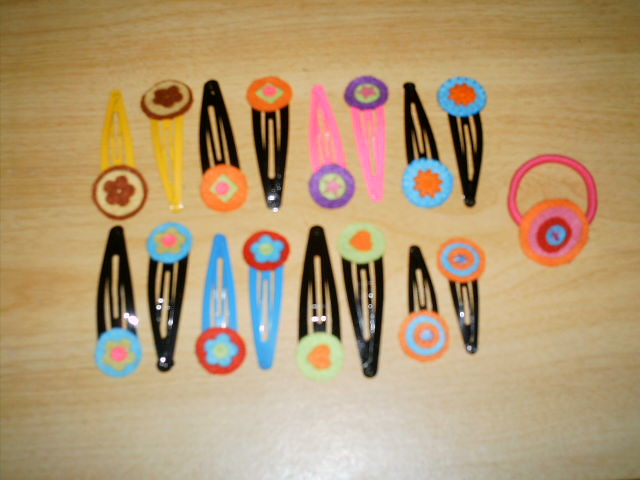The photograph features an overhead, slightly out-of-focus view of a light brown wooden table surface, showcasing its distinct wood texture. Arranged meticulously in a 3x8 grid pattern, the assortment of hair clips alternates between being placed upside down and right side up. The hair clips vary in color, including black, yellow, light blue, and pink, with their shiny surfaces suggesting they are made from either metal or plastic. Each hair clip is adorned with a circular end, which features a variety of intricate designs such as flowers, stars, hearts, and spirals. These designs are rendered in various color combinations like orange and light blue, orange and light green, blue and red, and purple and orange, contributing to the overall vibrant and visually engaging composition.